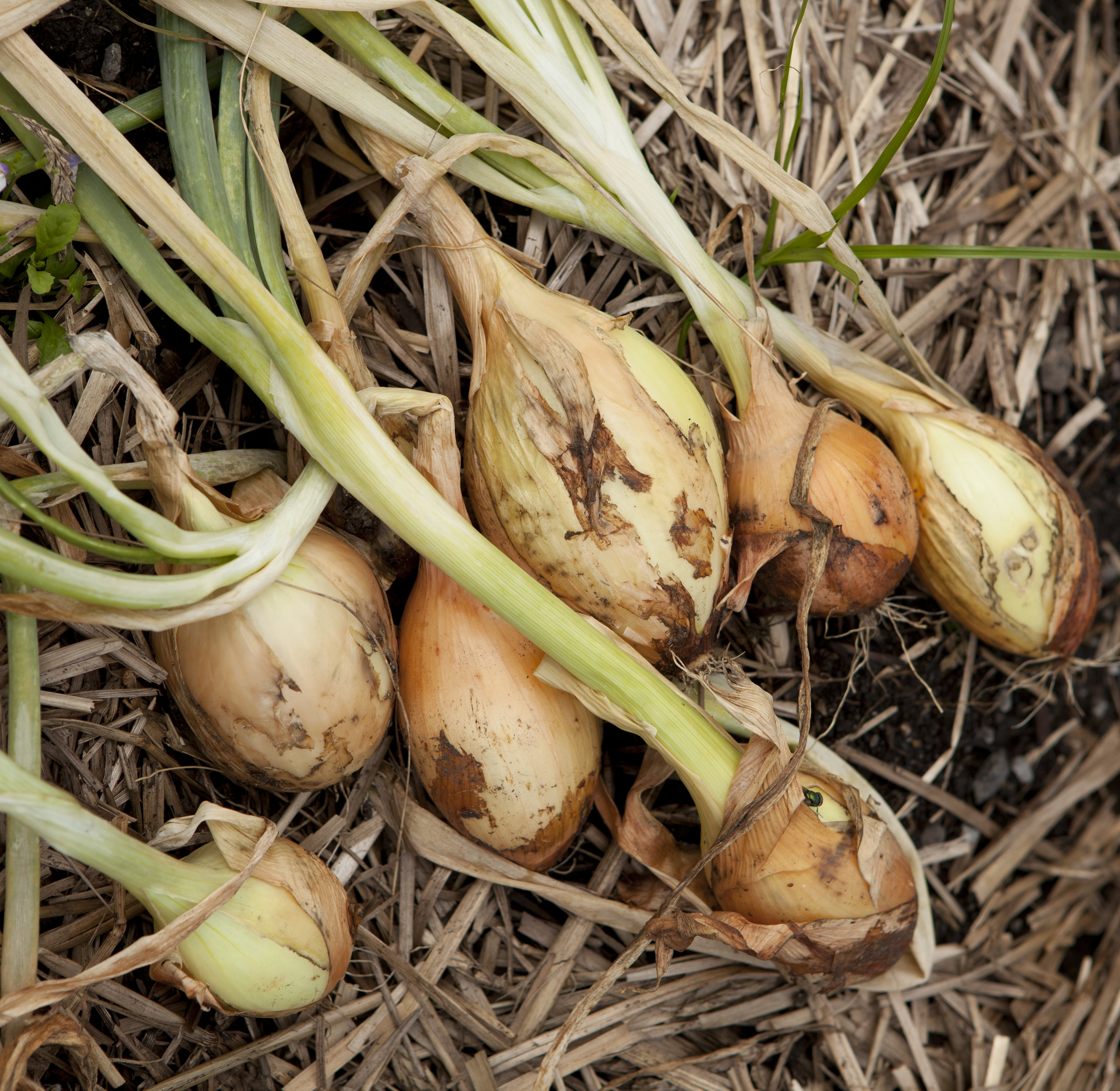This close-up photograph captures a cluster of recently harvested spring onions lying atop a bed of dried straw or hay. The onions, with their dark papery outer layers—some torn and some intact—exhibit bulbous white bases, still clinging to bits of brown earth. Pale green and yellowish shoots sprout from the bulbs, transitioning into long, vibrant green stems. The scene, set in an outdoor field, reveals the scruffiness of the roots protruding from the bottom ends of the bulbs, contrasting with the scattered straw and soil in the background.